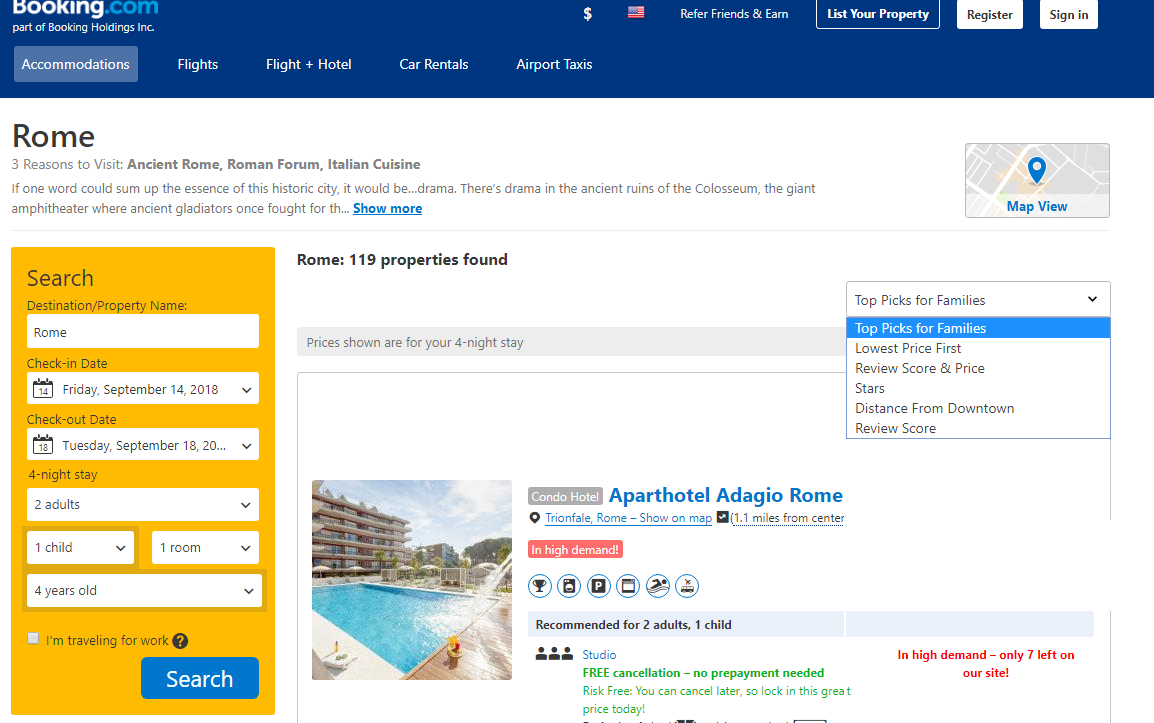Screenshot of Booking.com Website

This image captures a screenshot of the Booking.com website, a subsidiary of Booking Holdings, Inc. At the top of the webpage, there is a distinct blue banner featuring several navigational tabs, including "Accommodations," "Flights," "Flight + Hotel," "Car Rentals," and "Airport Taxis." Users can also find options to list their property, register, or sign in at the top of the site.

The specific page displayed in this screenshot is focused on available properties in Rome. Beneath the search bar, there is a section highlighting "Three Reasons to Visit Rome," mentioning Ancient Rome, the Roman Forum, and Italian Cuisine. The text suggests that if one word could encapsulate the essence of this historic city, it would be "drama," referencing the dramatic ancient ruins of the Colosseum, the giant amphitheater where gladiators once fought. A link labeled "Show More" is visible, offering further details.

The page also features a dropdown menu titled "Top Picks for Families," indicating 119 properties found. Prominently displayed is a single property listing for "Apart Hotel Adagio Rome," which is highlighted as being in high demand. The listing is recommended for two adults and one child, offering perks such as free cancellation and no prepayment needed, labeled as "risk-free" in green text.

On the left side of the screenshot, the search parameters are visible in a yellow box. The check-in date is set for September 14th, and the check-out date for September 18th, indicating a four-night stay for two adults and one four-year-old child in a single room. Additionally, there is an option to switch to a map view.